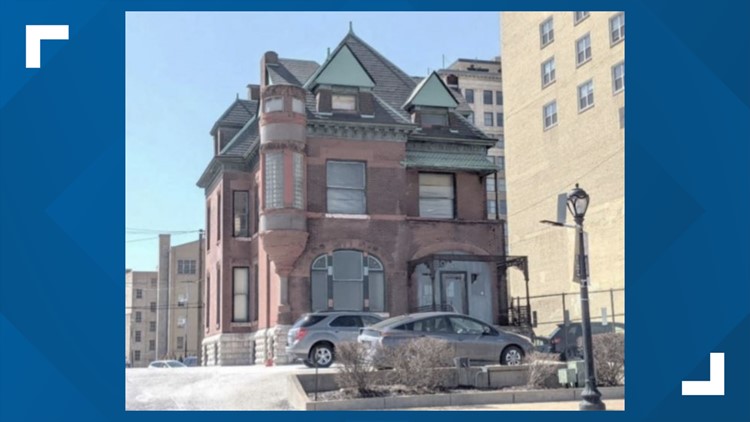The photograph depicts a city street scene dominated by a large, old red brick building with a turret and triangular roof points. This two-story structure features numerous arches and many windows. Parked in front of it are two silver vehicles, one likely an SUV and the other a sedan, alongside black lampposts. Adjacent to this building is an even taller, tan brick structure with multiple stories and rows of square windows beginning at the third floor. In the background, other tall buildings loom, suggesting a densely built cityscape. The scene is set against a slightly hazy, clear blue sky, with plenty of concrete surfaces visible for vehicles to navigate.